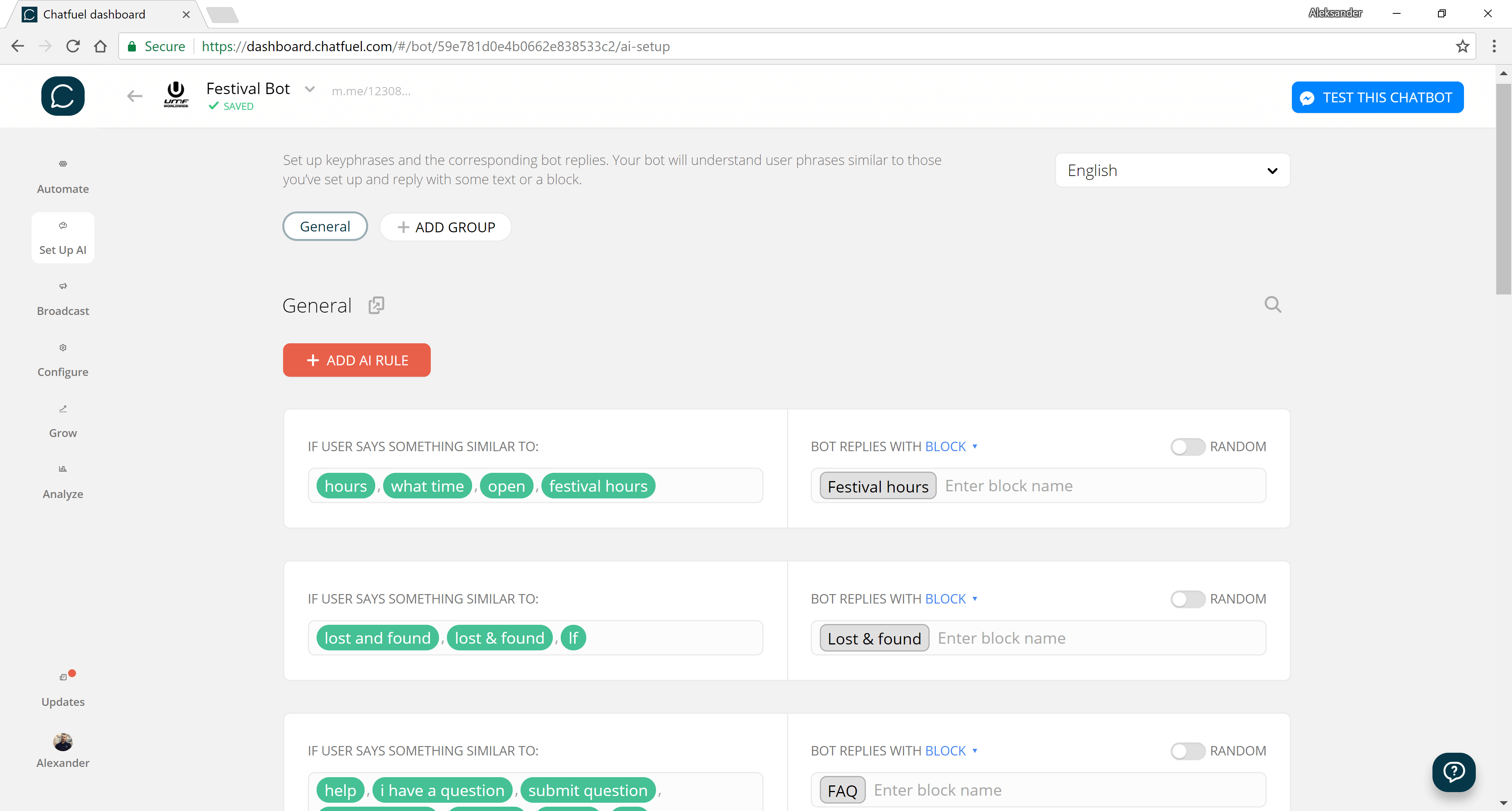The image displays a screenshot of a website featuring an off-white background. Positioned in the upper left corner of the screen, the title "chatwell-board" indicates the name of the application page. Below the title is the website's address bar, which includes a green padlock icon and the word "Secure" followed by "HTTPS" in green, with the remainder of the web address in black text. Below the address bar, the text "festival board" is visible in black. On the left side of the web page, a vertical menu lists various options and functions, including "automate," "set up," "AI," "breakfast," "configure," "grow," and "analyse." The right side of the image shows more of the web page content, featuring a prominent red button labeled "add AI role" in white text.